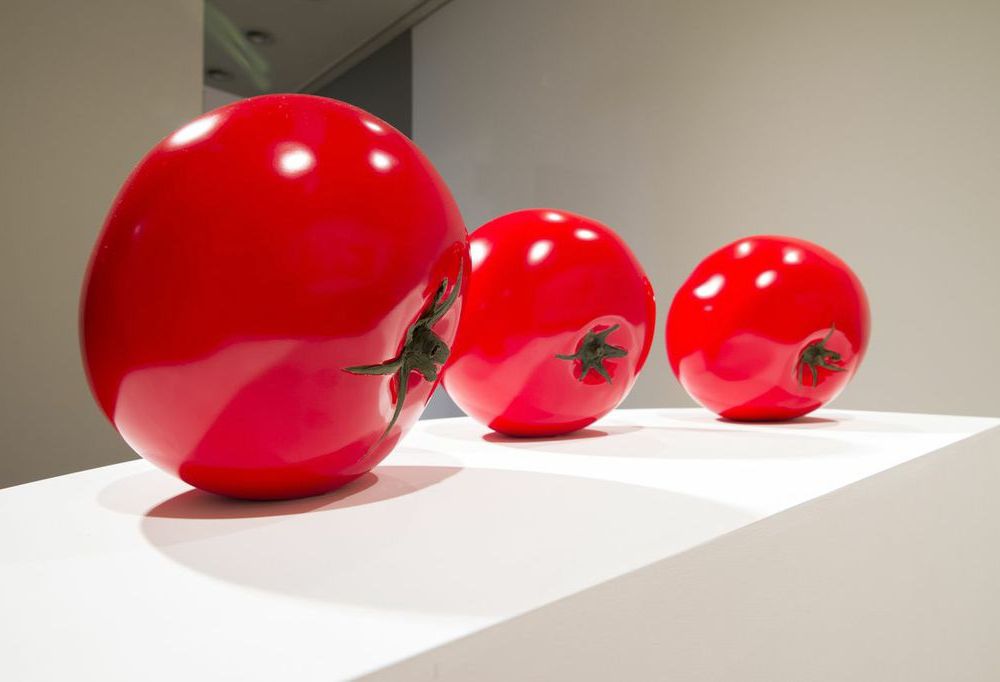This photograph captures a sculpture of three bright red, uniformly shaped tomatoes displayed on a white, rectangular platform. The tomatoes, which appear to be made of blown glass or plastic, are incredibly shiny and perfect in their form, reflecting overhead lights and casting spherical shadows on the pristine white base. The tomatoes are positioned side by side in a staggered line, with their green stems and leaves facing outward to the right. The surrounding room is stark white with minimal detail, likely part of a museum exhibit as suggested by the dedicated lighting focused on the sculpture. The environment lends an impression of perfection and uniformity, reinforcing the artificial nature of the tomatoes. The image’s plain background and lack of text highlight the simplicity and elegance of the display.